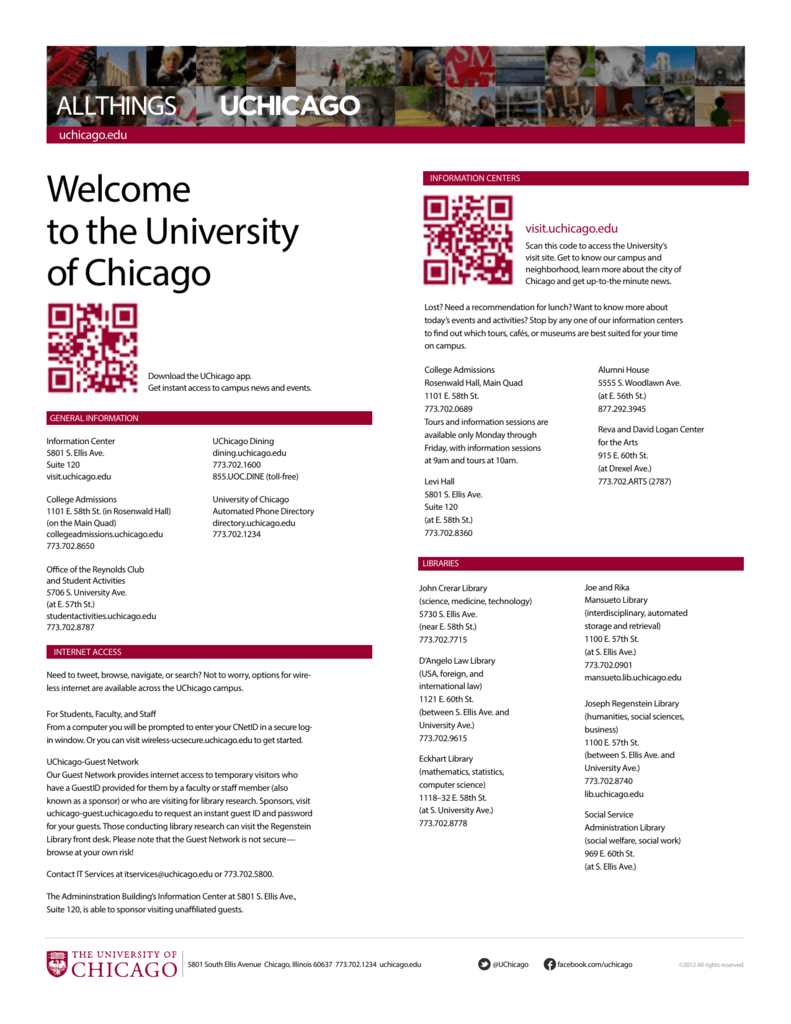This is a vertical rectangular image designed as an advertisement for the University of Chicago. The top section features a collage of various photographs seamlessly arranged next to each other, creating a dynamic visual header. Overlaid on the collage in bold white text are the words "All Things Chicago."

Beneath this collage, a thin burgundy border contains the text "uchicago.edu" in white, serving as the university's web address. Directly below this border is the main informational section presented in large black print. It begins with a welcoming message that reads, "Welcome to the University of Chicago." This section also includes a prominent QR code with a prompt encouraging viewers to "Download the UChicago app" to gain instant access to campus news and events.

The body of the image is divided into four main sections of information:
1. **General Information**: Provides key details about the university.
2. **Internet Access**: Guidelines and information on accessing the campus network.
3. **Centers** (upper right): The text is partially obscured, but it suggests information about various university centers, complete with another QR code.
4. **Libraries**: Offers detailed information about the university's libraries and their resources.

At the bottom, a thin line demarcates this extensive information from the footer. The footer includes essential contact details, stating "The University of Chicago," followed by the university’s physical address and the link to its Facebook page.